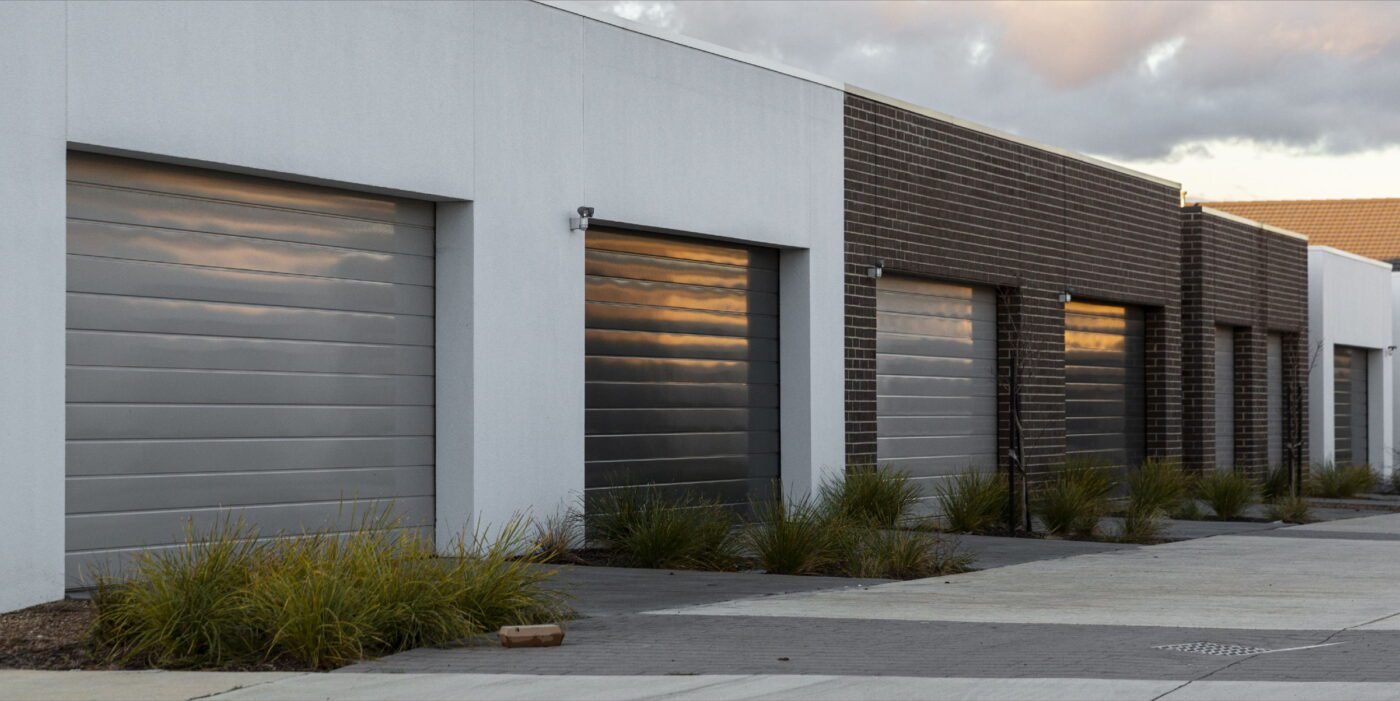This image showcases the exterior of a long, large storage facility captured at an angle. The structures alternate between sections of gray and black brick with white grout, giving it a visually striking appearance. The buildings feature garage-style accordion doors that also alternate in color between light gray and dark gray. The foreground is a light-colored concrete area, resembling a spacious sidewalk. In front of each of these garage doors are neatly maintained small grass patches with symmetrical green plants, adding a touch of greenery to the scene. Each section also has a light fixture, positioned beside the garage doors, highlighting the facility's layout and structure.